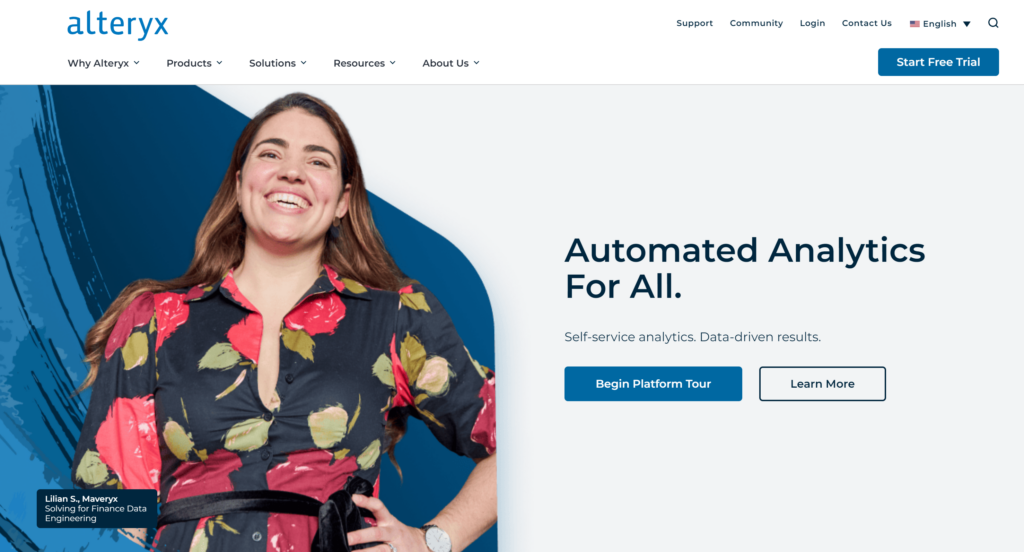This image captures the front page of the Alteryx website in meticulous detail. At the top left corner, the Alteryx logo is prominently featured, spelled out as "Alteryx" in bold, lowercase blue letters against a white backdrop. Directly below the logo, the navigation menu consists of five subsections: "Why Alteryx," "Products," "Resources," and "About Us," each accompanied by a drop-down menu for additional options.

On the top right portion of the page, several essential links are displayed: "Support," "Community," "Login," "Contact Us," and a language selection button labeled "English" with a drop-down menu. A search bar is also conveniently located in the top right corner for easy access.

Beneath the navigation bar is a prominent blue button with white text reading "Start Free Trial." The main body of the webpage features a grey background adorned with a striking graphic of a woman positioned behind a digital paint stroke. In the bottom left corner of this graphic, her name and position are displayed on a black rectangle.

Centered below this visual element is the tagline "Automated Analytics for All," rendered in large blue letters. Underneath, a subheading in smaller blue letters reads "Self-Service Analytics, Data-Driven Results." Completing the layout are two buttons at the bottom: a blue button on the left inviting users to "Begin Platform Tour" and a white button on the right offering the option to "Learn More."